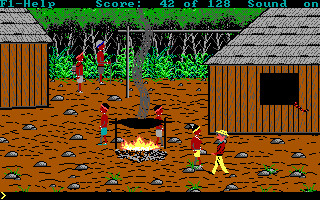This is a detailed screenshot from a video game, displaying a vibrant village campground scene. At the very top of the image, a black banner reads “F1-HELP” on the left, “score: 42 of 128” in the middle, and “sound on” towards the right, all in blue text. The foreground is marked by a thick black line with a yellow greater than symbol on the far left side.

Dominating the scene are two wooden huts on either side of the image. The hut on the left and the hut on the right both feature vertical wooden slats and gray, slightly thatched roofs. A distinguishing feature of the hut on the right is its black, square window. Scattered uniformly across the dark orange ground are small rocks, adding texture to the environment.

Central to the image is a fiery campfire, yellow and red flames dancing beneath a black cooking pot emitting smoke. Stones encircle the fire pit, creating a makeshift hearth. Beside the fire, two Native Americans, dressed in loincloths and head coverings, tend to the food. Their reddish skin glows in the firelight. There are three additional Native American men, similarly dressed, positioned around the scene—some in the background near crops that are meant for growing.

Adding to the cultural blend, a man with yellow pants, a brown jacket, and a yellow hat stands nearby, seemingly interacting with one of the natives. This man has pinkish skin and stands out distinctly against the native villagers. Behind him, another building features a thatched roof and similar construction as the other huts.

Green branches and whitish tree trunks can be glimpsed at the top, hinting at the surrounding nature. The scene combines elements of daily life, interaction between diverse characters, and a setting rich in detail and atmosphere.